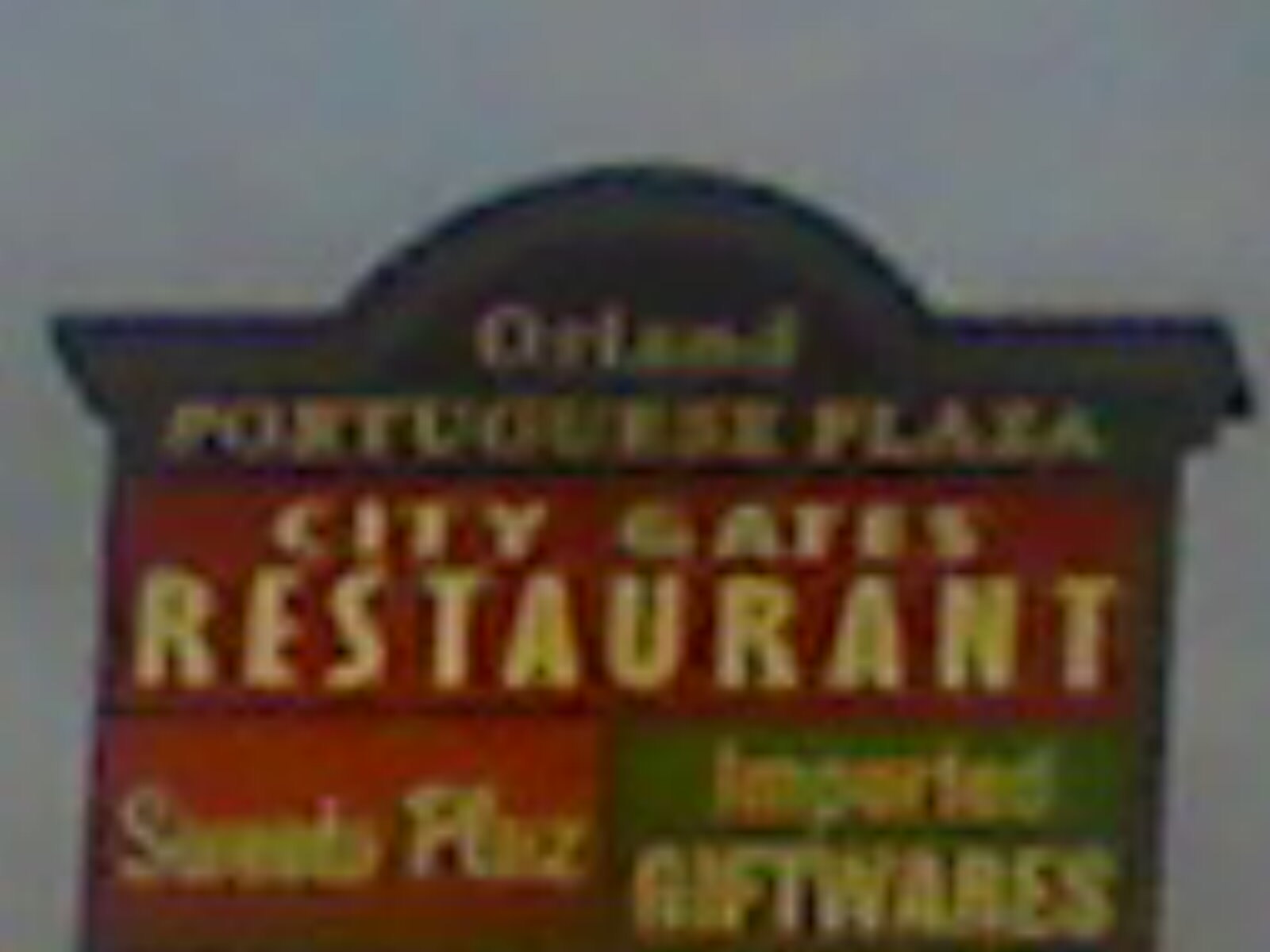This is a square color photograph capturing a very blurry and low-resolution sign situated against what appears to be a gray background, possible bits of blue suggesting the sky. The sign, dominating almost two-thirds of the photograph, features a straight top and a semicircular middle section. The topmost part of the sign, which is green, reads "Orland Portuguese Plaza" in white lettering. Directly below, on a thick red strip, the white text proclaims "City Gates Restaurant." The lower portion of the sign is divided into two sections: the left section has an orange background with unclear yellow writing—possibly "Sans Place" or a similar name, while the right section is green with yellow letters spelling "Imported Giftwares." All the text on the sign is either yellow or white, which contrasts against the different colored sections of the sign. The overall image is very grainy, making some of the finer details difficult to discern.